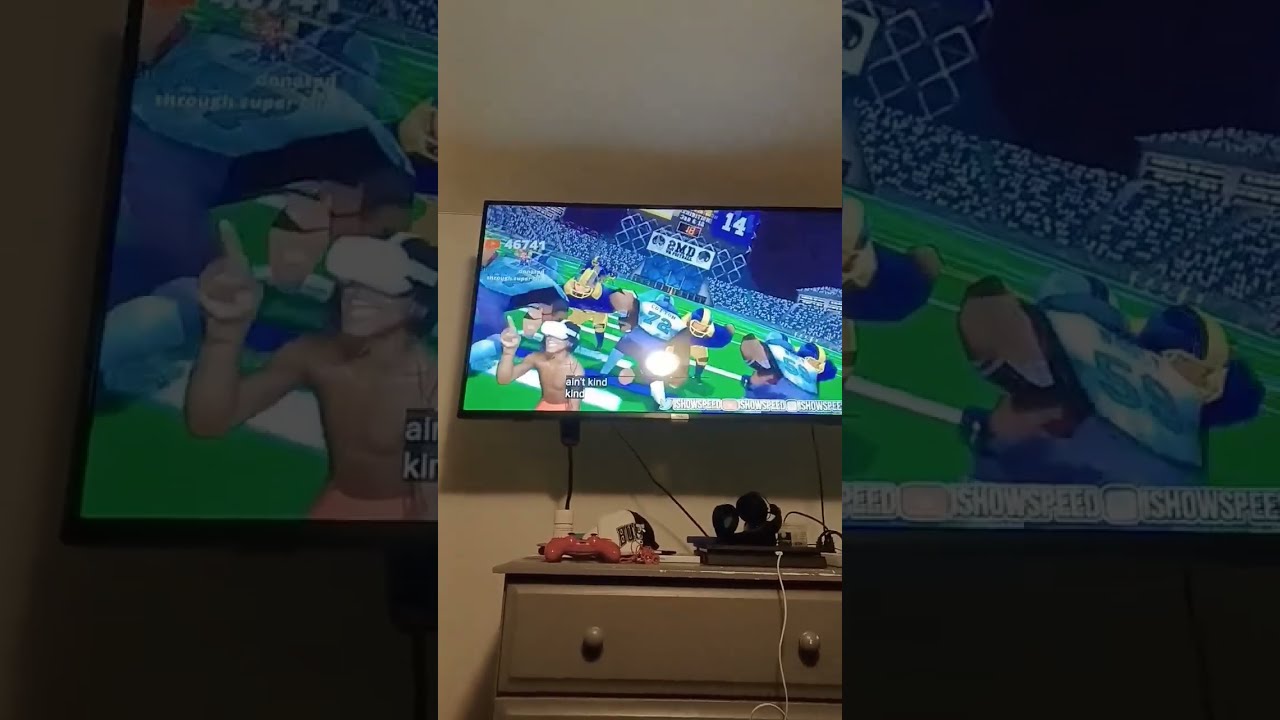This photograph features a television mounted on a gray drywall wall in a residential setting. The TV is displaying a video game, possibly a sports game, with vibrant blue, green, and white hues depicting a sports stadium filled with cartoonish characters. Beneath the TV, a brown dresser with a drawer bearing two knobs on each side serves as a stand for various objects. On top of the dresser, a slim PlayStation 4 console is connected with black and white wires, and a red video game controller is positioned alongside it. The image was taken vertically with a cell phone, and the background is a faded, zoomed-in version of the same scene, emphasizing the focal area with the TV and dresser. Several other miscellaneous items can also be spotted on the dresser's surface.